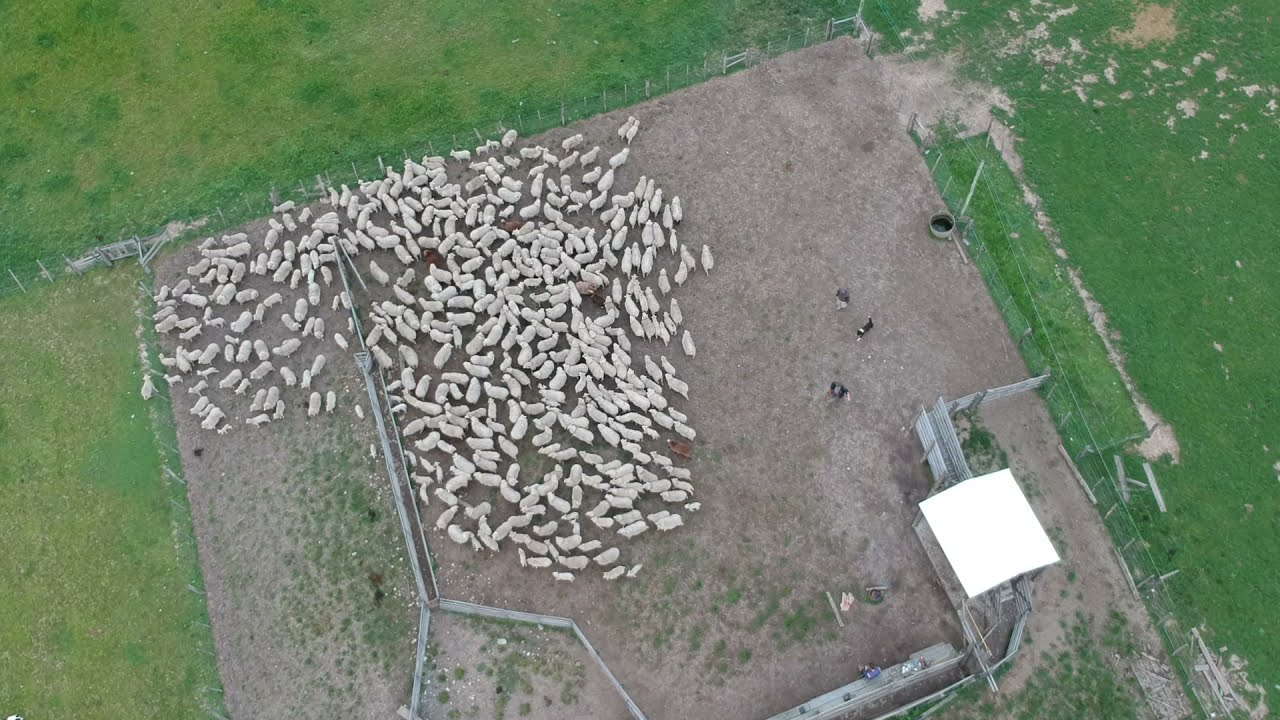This aerial image, likely captured by a drone, depicts a section of a farm highlighting a stark contrast between the lush greenery outside and the predominantly dirt-filled fenced-in pen. The pen, which appears to be divided into a larger and smaller segment with an open gate connecting them, houses a large congregation of animals. Predominantly white, these animals seem to be sheep, though there might also be a few goats and possibly dogs, as suggested by the presence of smaller, black-and-white creatures. Concentrated mostly in the middle area of the larger enclosure, with some moving towards the smaller section, these animals are surrounded by various farm structures and features. Notable among them are a small covered barn area, water barrels, and long troughs positioned within the pen, providing sustenance and shelter.